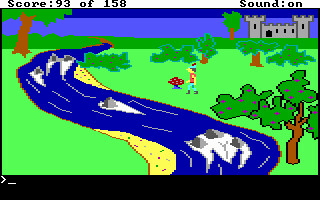This image is a low-resolution screenshot from a retro video game, characterized by its 8-bit, pixelated graphics. In the upper left corner, a black bar displays "Score: 93 of 150" in white text, while "Sound: On" is noted on the upper right. The center of the image features a blue river winding from the bottom toward the top, adorned with rocks that create a white-water effect, indicating movement. In the lower right corner, there's a small tree or large bush bearing red berries or apples. A more prominent tree is situated in the upper left. A grey castle dominates the upper right background, accompanied by additional trees and bushes. A lone figure, dressed in a red top, blue bottoms, and black boots, stands to the right of the river, near a red mushroom, looking off toward the left. A DOS-like command prompt is visible at the bottom of the screen, reinforcing the game's vintage aesthetic.